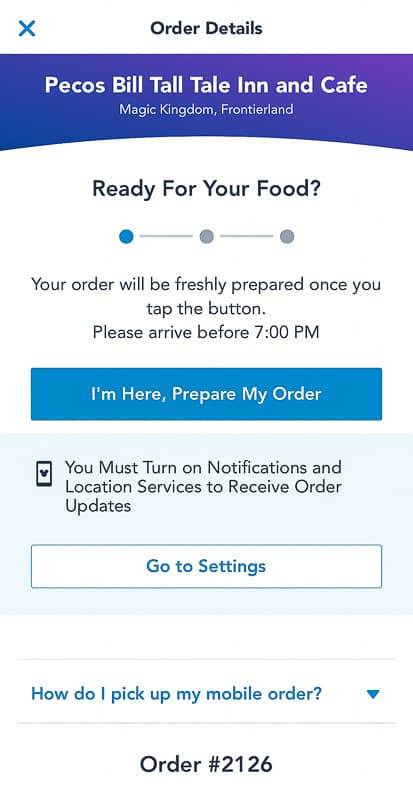This image is a screenshot of order details taken from a phone. At the very top, in small lettering, it reads "Order Details." Below this, set against a bluish-purple banner, is the text "Pecos Bill Tall Tale Inn and Cafe, Magic Kingdom, Frontierland."

The majority of the image is set against a white background, prominently displaying the message, "Ready for Your Food," followed by three dots indicating the progress of the order. Below this, the text advises, "Your order will be freshly prepared once you tap the button. Please arrive before 7 p.m."

A large blue button with bold lettering states, "I'm here, prepare my order." Further down, there is a smaller, light blue window emphasizing the necessity to "Turn on notifications and location services to receive order updates." Beneath this, there is a button labeled "Go to settings."

At the bottom of the page, the text inquires, "How do I pick up my mobile order?" next to a collapsible, clickable menu arrow for more information. Finally, at the very bottom, the order number is displayed: "Order Number: 2126." The entire screenshot maintains a clean, white background for ease of readability.